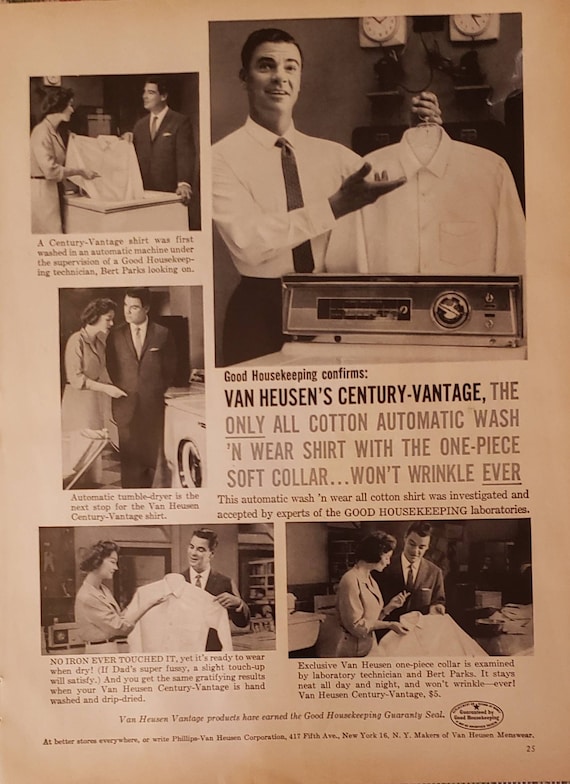The sepia-toned, black-and-white image resembles a vintage magazine or newspaper advertisement prominently displaying a Van Heusen Century Vantage shirt. The ad, found on page 25, features various photographs and detailed paragraphs, emphasizing the shirt's unique qualities. It highlights that the Century Vantage shirt, an all-cotton garment with a one-piece soft collar that won't wrinkle, was first tested in an automatic washing machine under the supervision of a Good Housekeeping technician named Bert Perks. The shirt also underwent testing in an automatic tumble dryer, with no iron used, emerging ready to wear. The Good Housekeeping laboratories confirmed its durability and ease of care, noting that even minimal touch-ups would satisfy the most meticulous users. The ad’s vintage aesthetic, reminiscent of the 1950s, showcases multiple steps including a woman and her husband demonstrating the shirt’s care process, reinforcing its convenience and quality.